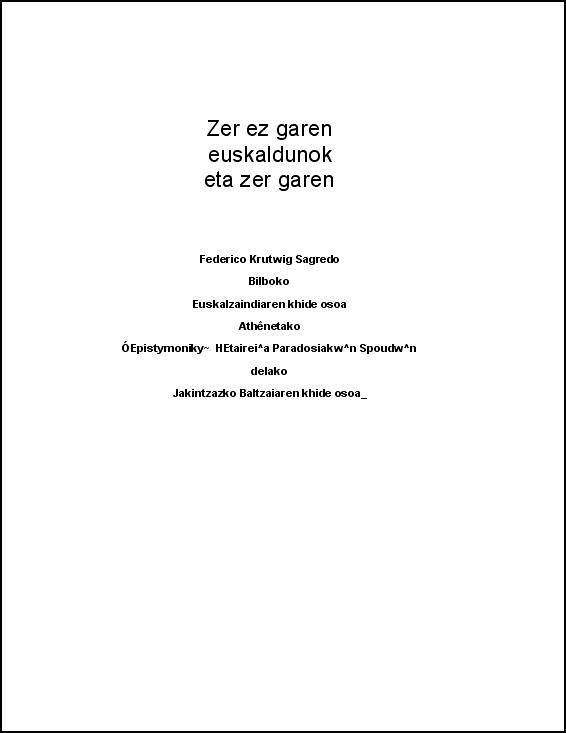The image features a rectangular, white background with a thin black border. The centerpiece of this composition is a block of centrally aligned black text, largely in a foreign language, consisting of three larger lines at the top followed by seven smaller lines below. 

The larger text at the top reads: "Zer ezin garen euskaldunak eta zer garen." Underneath this, separated by several blank lines, is a smaller yet bold section reading, "Federico Krutwig Sagredo," followed by "Bilbioko Euskalzainadiar en khide osoa," and "Athenetakoo OOE pistymoniky - Hetarei Paradisiakwn Spoudw." The final line in finer print reads: "delako Jakintzazko Baldaairen khide osoa -."

Overall, the minimalist design emphasizes the black text against the stark white background, with the text neatly centered within the frame.